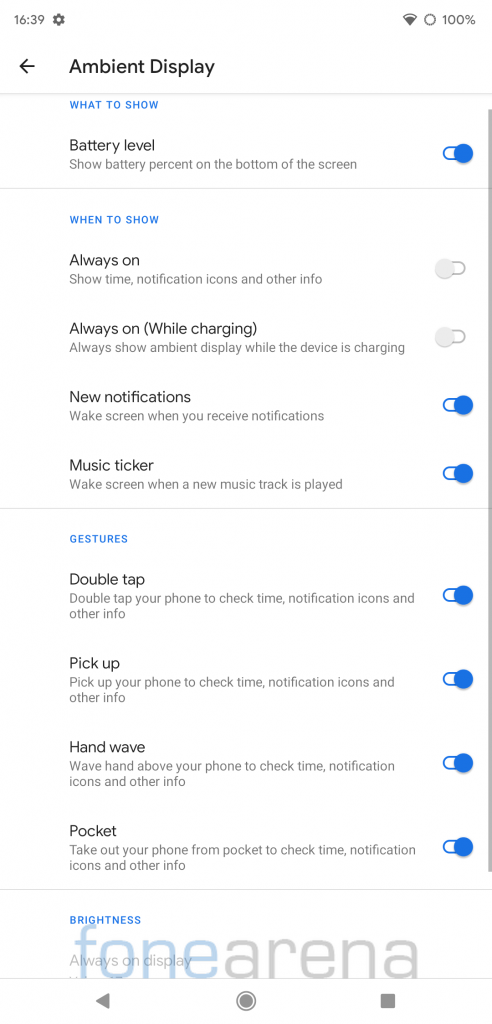The image depicts a detailed view of a mobile phone's settings, specifically focusing on the "Ambient Display" settings. At the top right corner, the phone's battery status is displayed at 100%, adjacent to a gray circle icon, and a Wi-Fi signal icon showing near-maximum strength. The current time, shown in the top left corner, is 16:39, with a gear icon to its immediate right. Centered at the top, the words "Ambient Display" are evident with an arrow pointing left beneath it, followed by a thin gray dividing line.

Under the heading "What to show," highlighted in blue text, the first option reads "Battery level," which is followed by the option "Show battery percent on the bottom of the screen." To the right of this text is a toggle switch set to the "on" position, indicated by its blue color. Another thin gray line separates this category from the subsequent section.

In the middle of the image, under the heading "When to show," there are four selectable options: "Always on," "Always on while charging," "New notifications," and "Music ticker." The final section, labeled "Gestures," provides four options for user interaction: "Double tap," "Pickup," and "Wave pockets." Each of these categories and options are clearly delineated for a structured and easy-to-navigate user experience.